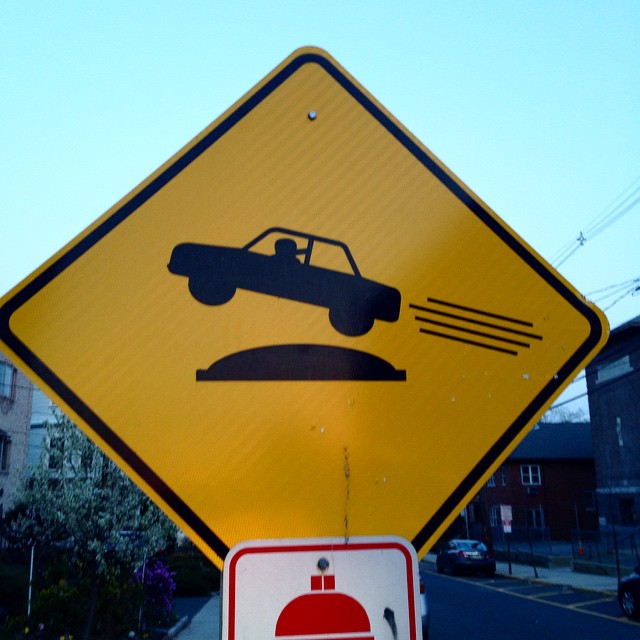The photograph features a distinctive diamond-shaped street sign captured against the backdrop of a neighborhood. The sign itself is a cautionary yellow, with a striking black silhouette depicting a car seemingly leaping through the air over a half-circle ramp. The car's dynamic leap is accentuated by motion lines trailing from its rear. Interestingly, the driver is clearly visible and notably wearing a seatbelt, adding a touch of realism to an otherwise whimsical scene that might evoke memories of the "Dukes of Hazzard."

In the background, a residential area comes into view, with structures that could be houses, apartments, or perhaps even churches. The right side of the road features a few parked, dark-colored cars, possibly dark gray. The sky overhead is a serene aqua, suggesting the onset of early evening or a sunset in progress. The overall ambiance of the image blends playful caution with the tranquil end of a day.